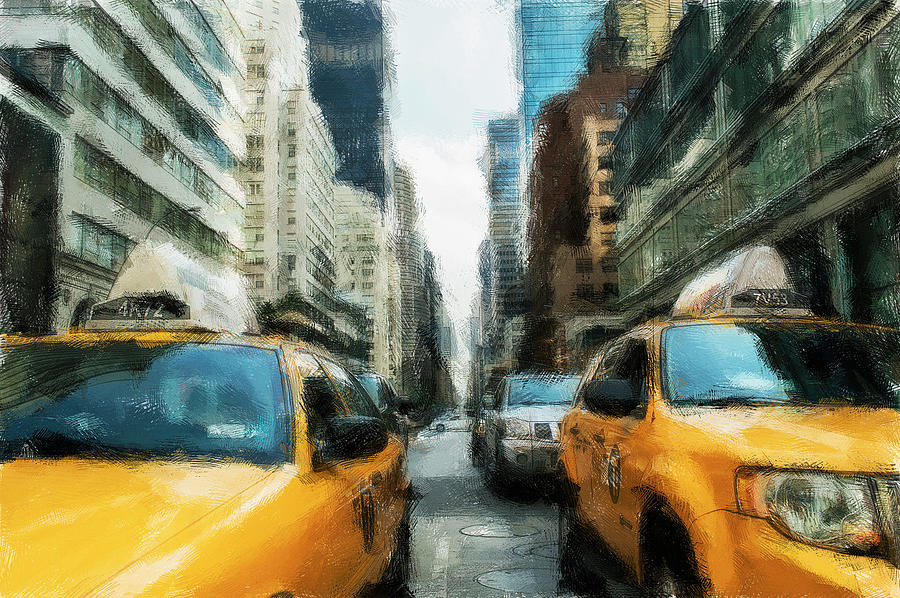The image portrays an artistic rendering of a bustling city street, likely in New York City, given the prominent presence of iconic yellow taxis. The artwork utilizes Impressionist techniques, featuring visible brush strokes and a rich blend of colors that imbue the scene with a vibrant, almost dreamlike quality. Centrally, the street, lined with towering high-rise buildings, divides the composition. These structures are adorned with uniformly-sized glass windows that reflect the overcast, cloudy sky, painted in subdued whites and grays.

In the foreground, two bright yellow taxis immediately catch the eye. One is positioned on the left, viewed from the side, while the other faces the viewer directly. Alongside these taxis, additional vehicles—a black car and a silver car—add to the sense of urban congestion. The overall scene captures the dynamic and hectic essence of city life through a blend of deliberate blurriness and vivid impressionistic details.